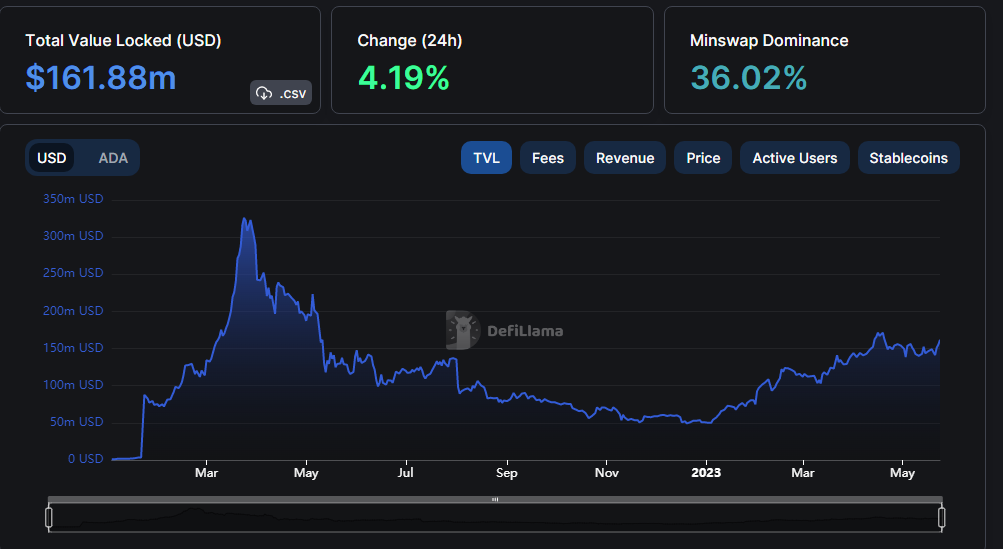The image, extracted from a webpage dedicated to stock or financial information, features a detailed black background. At the top left corner, white text reads "Total Value Locked (USD)," followed by labels such as "Change" and "24H." Additionally, "Minswap Dominance" is highlighted. Below these headings, numerical data shows "$161.88M" (likely indicating millions), a green "4.19%," and a teal "36.02%."

The line graph presented in the image charts data points from March, May, July, September, and November, spanning multiple years until March and May of 2023, where it abruptly ends. The y-axis of the graph measures in USD, ranging from zero to 350 million USD. The graph also includes "ADA" alongside "USD," indicating dual measurement units. The image provides a comprehensive visual representation of the financial data spanning over time.